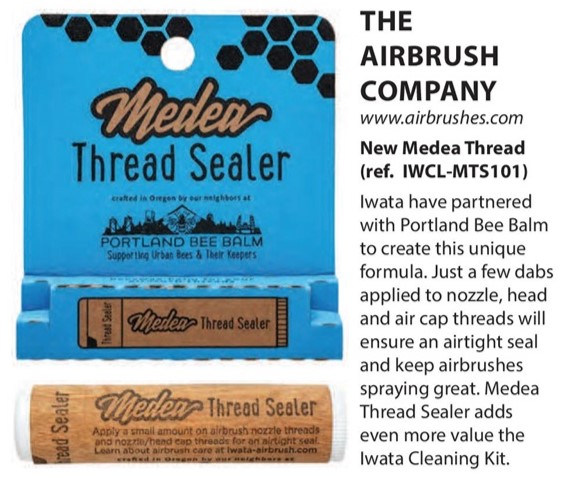The image showcases an advertisement for the Medea Thread Sealer, prominently featured in a blue packaging that reads "Medea Thread Sealer" and "Portland Bee Balm, supporting urban bees and their keepers." Crafted in Oregon by Portland Bee Balm, this product is designed for airbrush maintenance. A visual of the chapstick-like thread sealer tube is displayed, with instructions to apply a small amount to airbrush nozzle threads and nozzle head cap threads for an airtight seal. For further airbrush care instructions, a website is provided. On the right side of the image, the text highlights the Airbrush Company (www.airbrushes.com), announcing a new Medea Thread Sealer with a reference number IWCL MTS 101. It also mentions a partnership between Iwata and Portland Bee Balm to create this unique formula which ensures an airtight seal with just a few dabs, enhancing the performance of airbrushes. Additionally, the Medea Thread Sealer complements the Iwata Cleaning Kit, adding even more value for airbrush users.